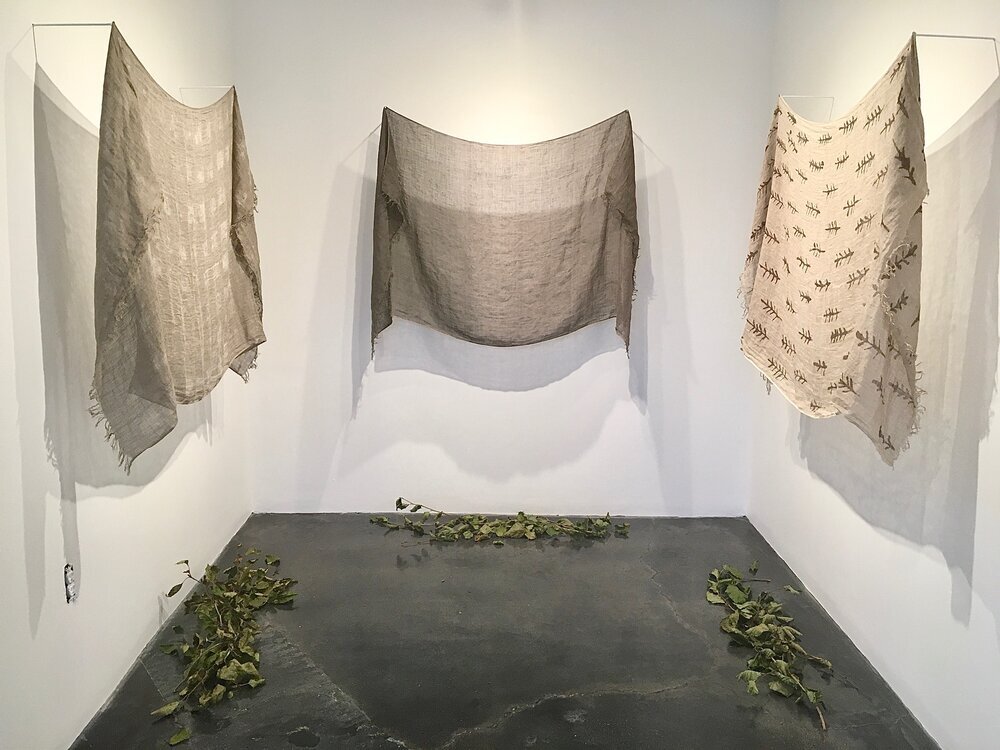The image captures an indoor scene resembling an art exhibit or installation. The color photograph depicts a room with three visible walls and a floor, where each wall hosts a hanging cloth or fabric. The fabrics are suspended from rods attached perpendicularly to the walls. The rightmost cloth is beige and adorned with a twig-like pattern, while the other two cloths are darker shades of brown or gray. Each hanging fabric casts distinct shadows on the walls behind them.

The flooring is a dark gray to black material, likely resembling black marble or concrete. Scattered on the floor beneath each fabric are piles of dried leaves, emphasizing a sense of decay or natural elements. An electrical outlet without a cover is visible on the left wall, subtly hinting at the room's practical background juxtaposed against its artistic presentation. This meticulous arrangement of hanging fabrics and leaf piles suggests a carefully curated art installation aimed at evoking thought or emotion through its minimalist and organic components.